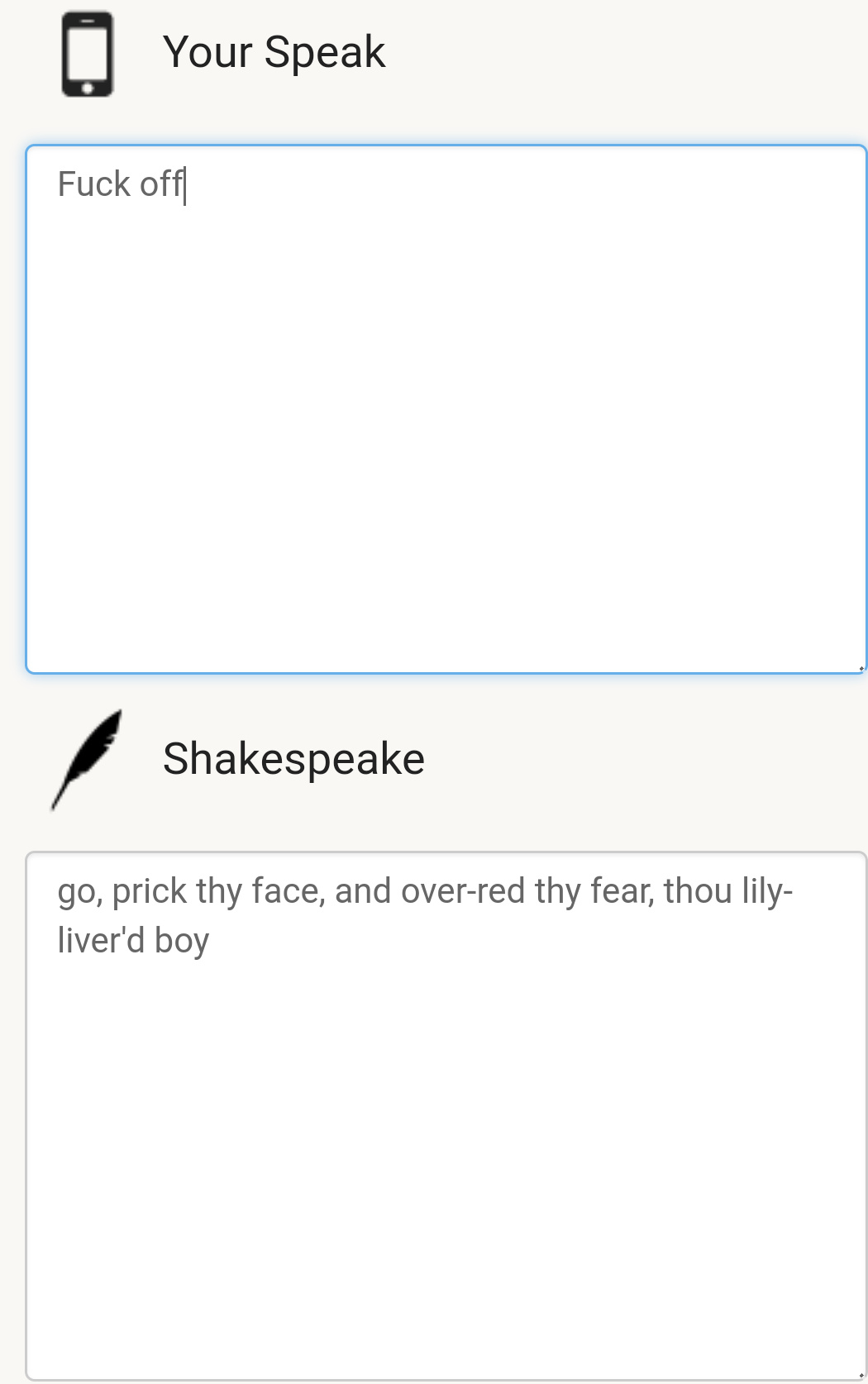This image features two open squares intended for text input. At the top, a small message sits within a square, while a larger sentence is positioned within the bottom square. The top square has a light gray background and includes a cell phone icon. Below this square is a white square outlined in blue, containing the text "Down below is a feather icon that’s black, and it just says Shakespeare to the right of that. Actually, Shakespeare." The bottom square, outlined in light gray, completes the visual with the message "That's the message outlined with a light gray square." This design effectively segments content into distinct areas for clearer communication.